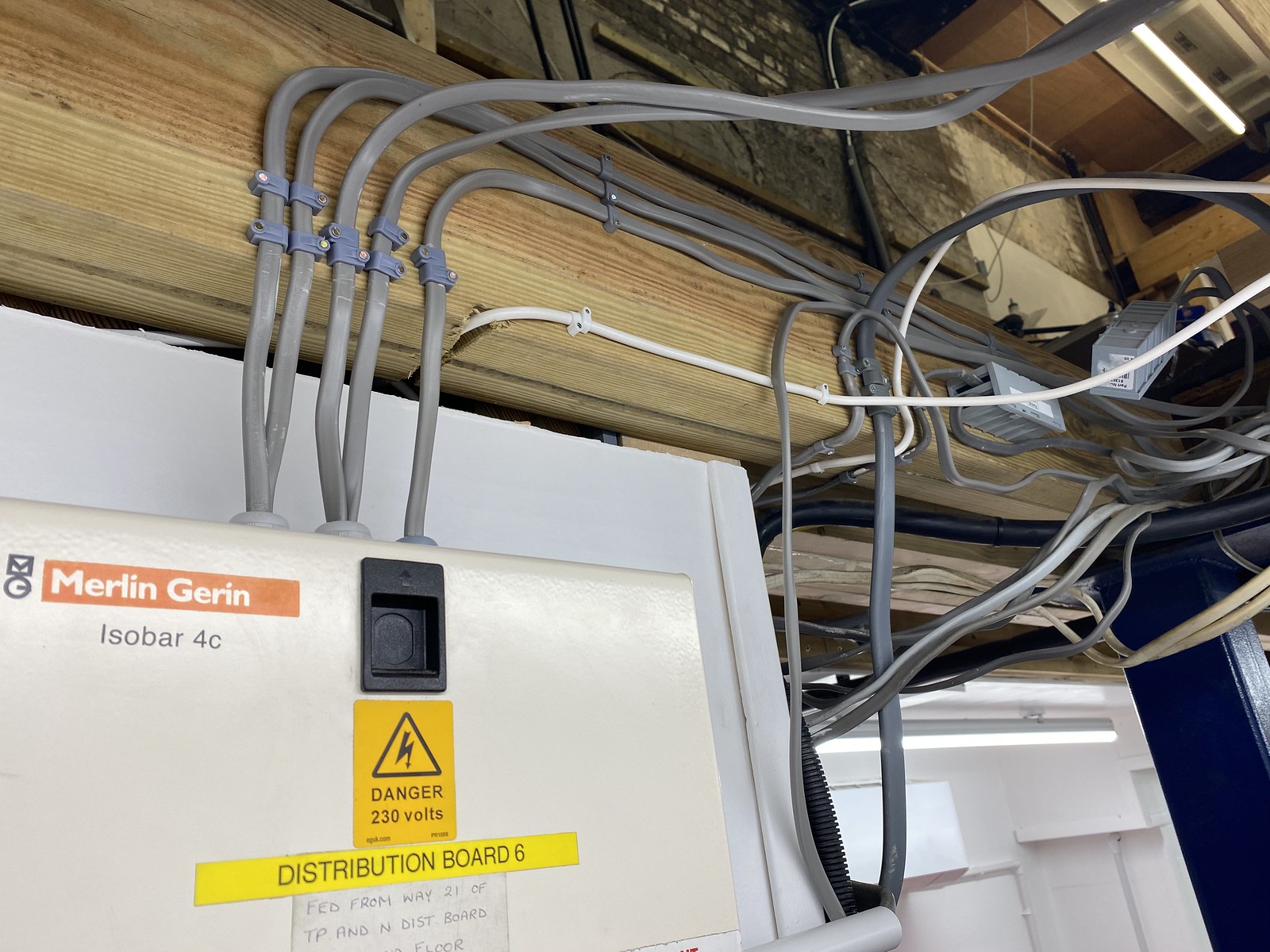The image shows an up-close view of the interior of a building, specifically highlighting an electrical setup. Prominently featured is a white rectangular electrical box attached to a tan-colored wooden support beam. Several thick gray and white cords are connected to this box, emerging from both its side and top. The box displays an orange rectangle with white lettering saying "Merlin Gerin, Isobar 4C." Below a black indented handle, there's a yellow label with black lettering displaying a black triangle with a lightning bolt and the warning "Danger 230 Volts." Furthermore, a white card affixed to the box reads, "February from May 21 of TP and N DIST board." To the right of this electrical box, smaller gray boxes and additional cords are visible, also attached to the beam and ceiling structure. Adjacent to this setup is a tall bluish square beam extending out of the frame, with a white wall beyond it. The building appears to have an attic-like or basement atmosphere, emphasized by the supporting beams and overall unfinished look.